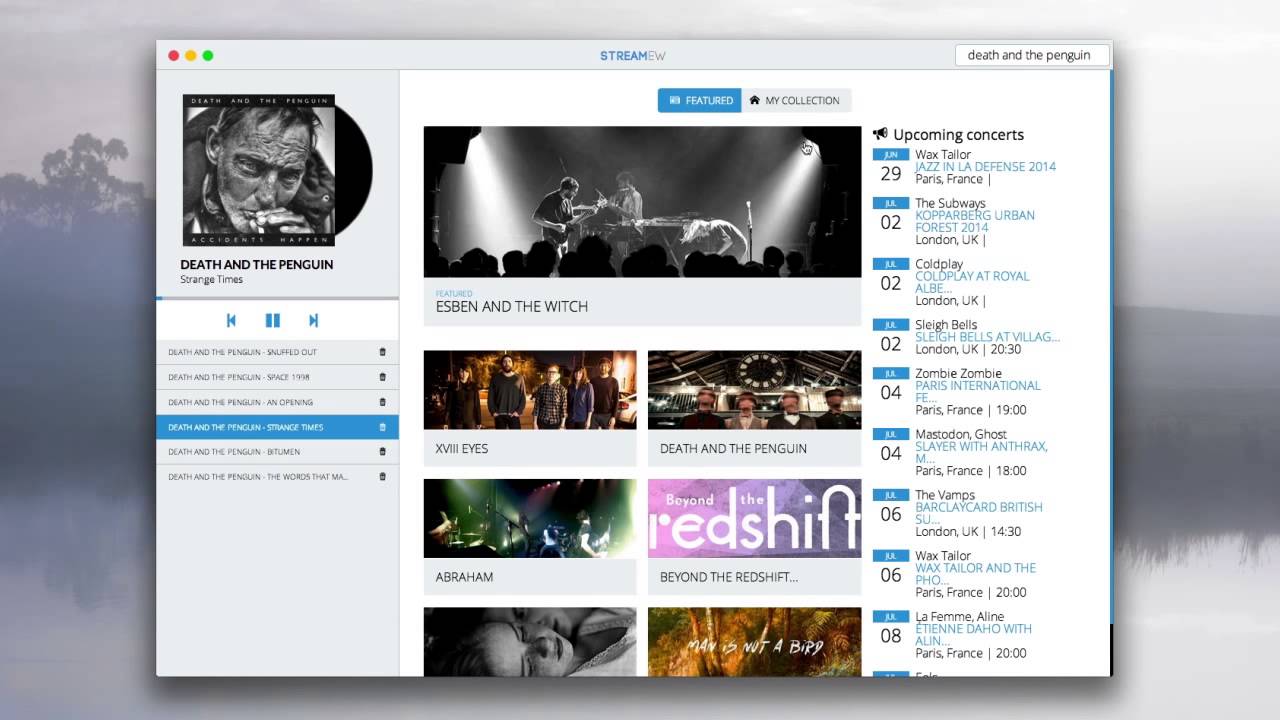This image is a screenshot from a music streaming website called "Stream New." The top of the image prominently displays the site's name. A search box near the top has been filled in with the words "Death and the Penguin," indicating that this is the artist being searched for. The search returns a black-and-white image of a man smoking a cigarette, likely the cover art for one of their albums, with the title "Death and the Penguin - Strange Times" underneath.

Directly below this, there is an interface that allows users to play content from this album. The main section of the page is populated with additional artists, shown in seven images down the center of the screen. Each image features either performance shots or posed pictures of different artists and bands, and clicking on these images will direct users to their respective content on the streaming site.

On the right-hand side, there's a section dedicated to upcoming concerts, displayed in a calendar format. The events listed span from June 29th to July 8th and include concerts in both Paris and London, suggesting a mixture of local and international events.

Overall, the screenshot gives a comprehensive look at the user interface of a music streaming platform, highlighting search functionality, artist-specific content, suggestions for additional artists, and a calendar of upcoming concerts for multiple locations.